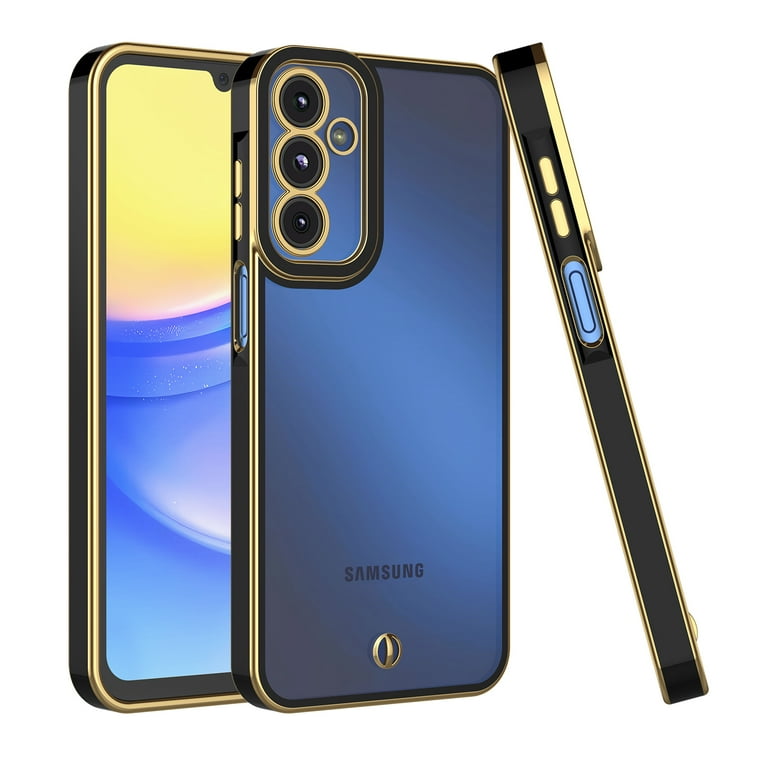This detailed photograph showcases a Samsung Galaxy smartphone from multiple angles, with each perspective artfully superimposed to provide a comprehensive view of the device. In the foreground, the front-facing view of the phone reveals a screen adorned with yellow, pink, blue, and darker blue hues, framed by a gold bezel that adds a touch of elegance. The phone's rim is black, enhancing the visual appeal. Partially obscuring the screen, another phone is laid atop it, presenting the backside which features a navy-blue color and the Samsung logo prominently displayed at the bottom. This rear view of the phone highlights a sophisticated camera setup with three stacked lenses, encircled by a gold trim and surrounded by a black rim. Propped against this rear view is the side profile of the phone, revealing its thin, sleek design reminiscent of an iPhone. The side view showcases a distinctive button arrangement, with gold volume buttons and a blue power button, all set against a black and gold case. This multi-angled presentation vividly captures the intricate design and aesthetic details of the Samsung Galaxy smartphone.